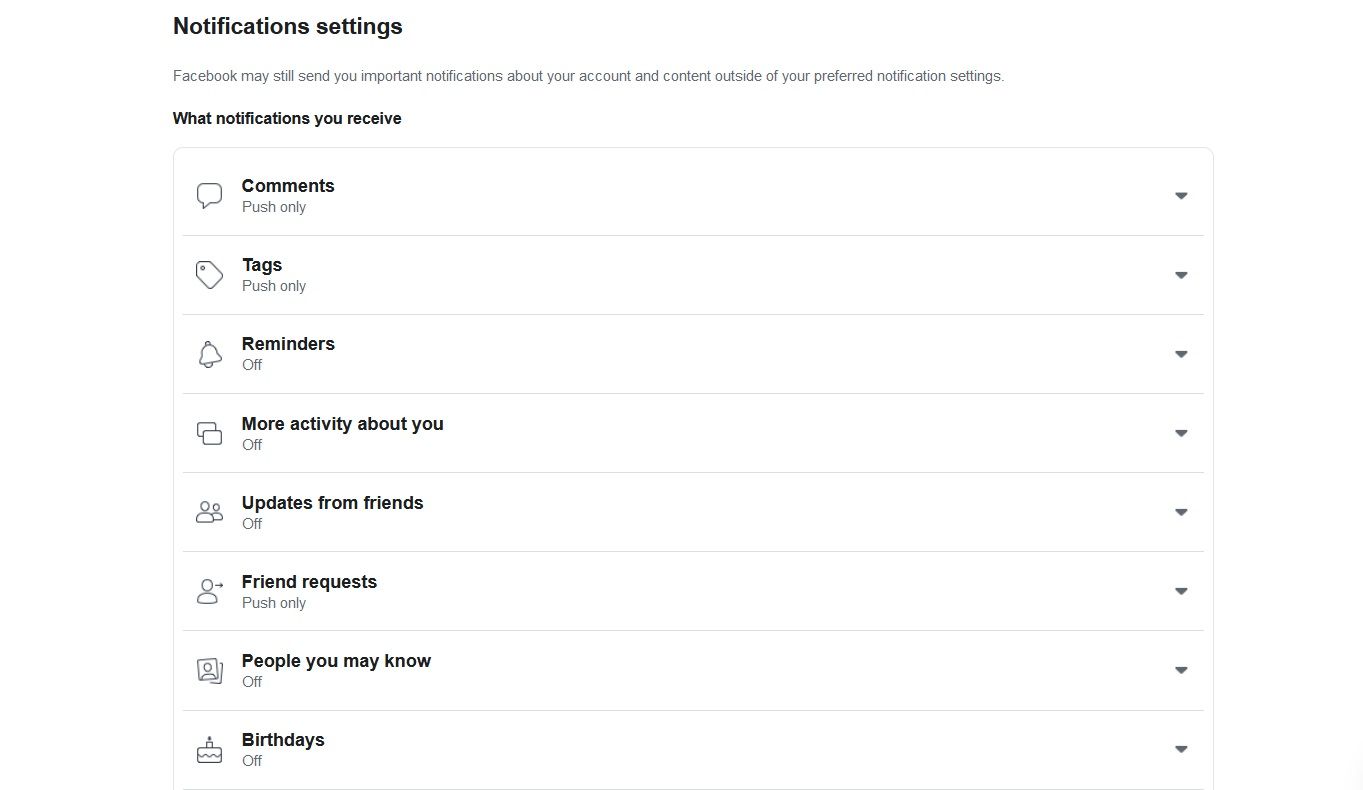The image displays a white text box organized in a list or table format, segmented by thin gray lines. At the top left corner, bold black text reads "Notifications Settings." Below this heading is a description stating that "Facebook may still send you important notifications about your account and content outside of your preferred notification settings." The text also indicates "What notifications you receive," followed by a series of boxes that list different notification options, each accompanied by an icon on the left side.

The categories of notifications, presented in bold black text from top to bottom, are as follows:
- Comments (Push only)
- Tags (Push only)
- Reminders (Off)
- More activity about you (Off)
- Updates from friends (Off)
- Friend requests (Push only)
- People you may know (Off)
- Birthdays (Off)

To the right of each category, there are small gray arrows arranged vertically, pointing downward, indicating that a drop-down menu can be accessed to change the settings for each notification type.